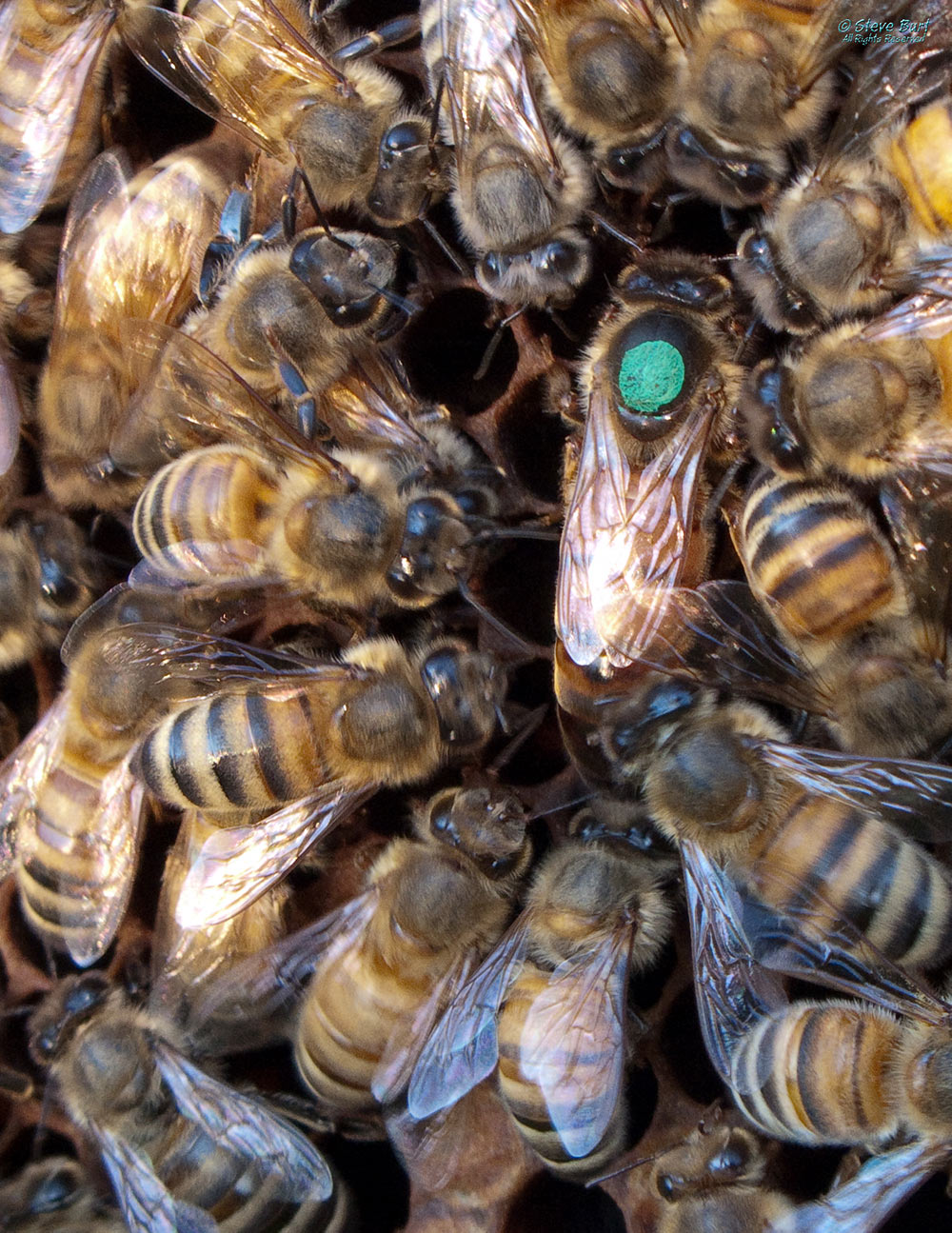This close-up, horizontally oriented nature photograph captures a bustling beehive teeming with honeybees. The bees, slightly furry with yellow and black striped bodies and big black eyes, are densely clustered across the frame, creating a frenetic mosaic of busyness. Central to the photograph is a honeybee marked with a small, bright emerald green dot on its back, likely indicating its role as the queen bee, despite being similar in size to the others. This marking, possibly used for identification or tracking purposes, draws the viewer's eye amidst the swarm. The bees are surrounding the queen, many with their wings folded, engaged in various activities essential to the hive's function. Bits of the honeycomb, dark brown and hexagonally patterned, peek through the mass of bees, further emphasizing the industrious nature of these insects. The overall scene suggests a snapshot of a lively and active beehive, possibly during spring or summer, with bees tending to their queen, depositing nectar, and maintaining hive operations.